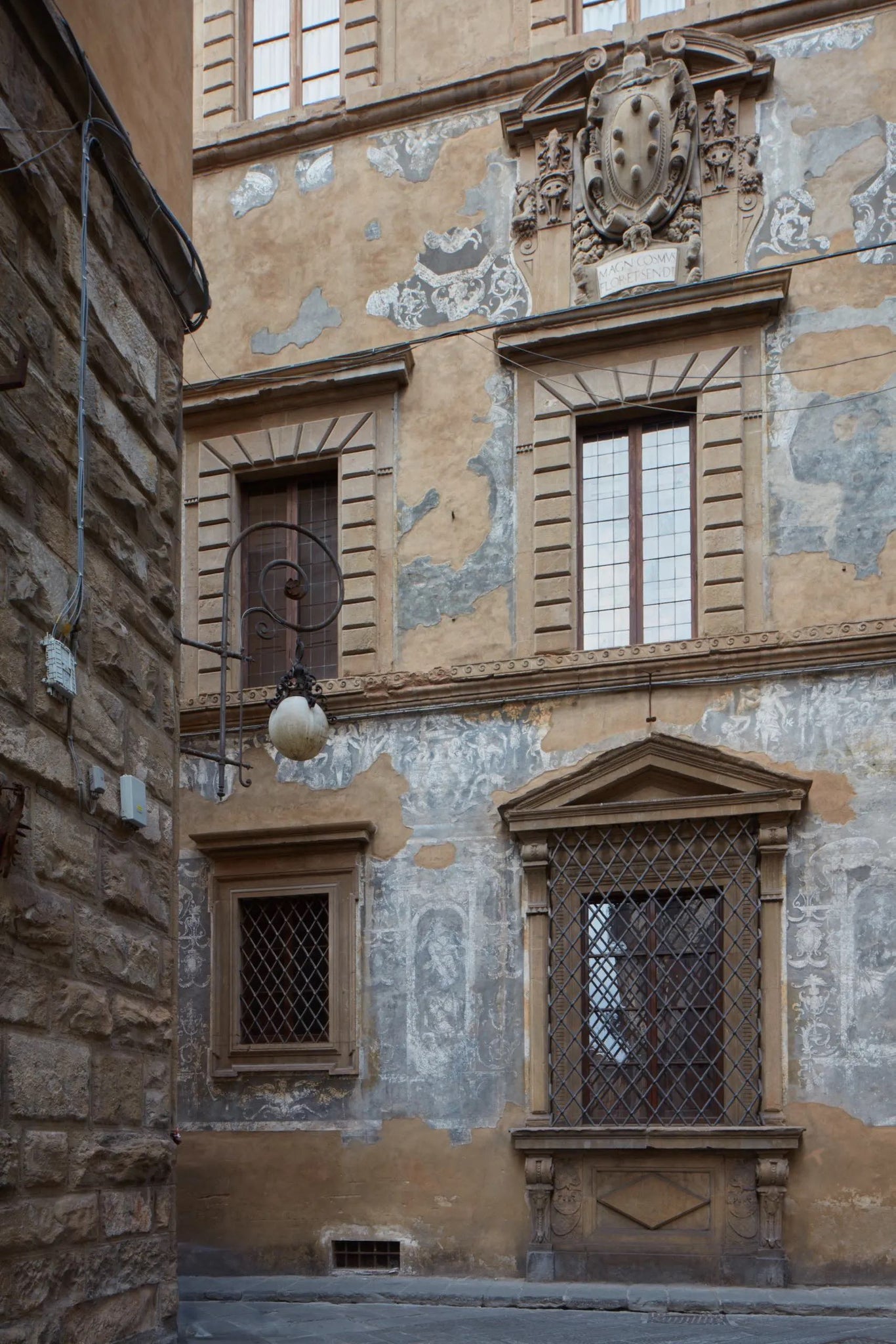This vertical, rectangular color photograph captures the facade of the historic Hotel Bavaria in Florence, Italy. The building exhibits a classical European architectural style and is primarily constructed from concrete, accented by aged beige stucco and gray with white motifs. The facade features several ornate window openings, and the bottom windows are protected by steel mesh coverings, topped with short pediments and supported by ledges underneath. Visible in the upper central area is a molded coat of arms, which appears three-dimensional and includes a shield adorned with dots and a Latin inscription on a curved plaque beneath it, though the text is illegible due to deterioration. Another building to the left is made of stone, and its facade includes a peculiar lamp with a curved wrought iron top and a round white light. The overall scene showcases a blend of decaying grandeur and intricate detail, capturing the essence of European aesthetic and aging architecture.